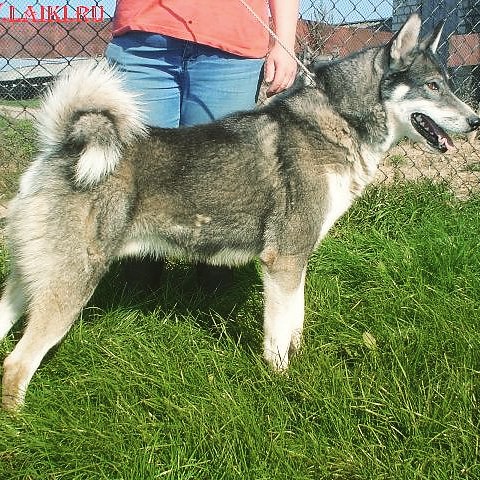The image captures a striking dog that bears a fierce and ferocious resemblance to a wolf, identified by its signature husky traits such as a black-and-white or brownish-blackish coat, pointed ears, and a curled tail. The husky mix, with its sharp teeth and intense gaze directed forward, stands on a vibrant patch of green grass. Only one side of the dog is visible, emphasizing its majestic profile. Partially obscured by the dog, the owner is partially visible, wearing a reddish-orange t-shirt and blue jeans, holding the leash. They stand in front of a metal fence with some low-rise buildings in the distant background. The dog's collar and the minimal visible part of the owner's attire add a brief but essential context to this dynamic and commanding image.